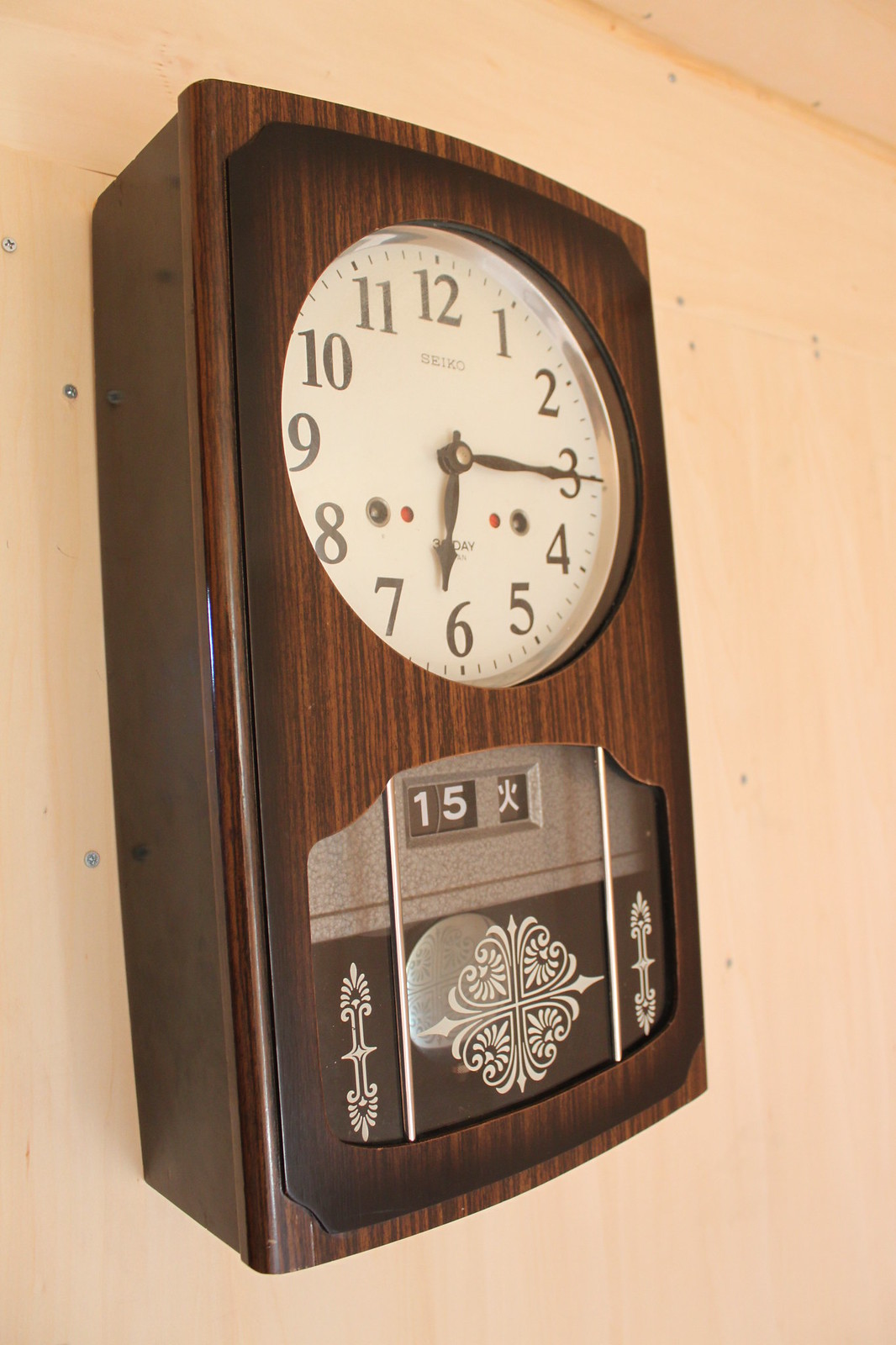This photograph captures a clock mounted high on a wall painted in a very dull, matte-finished pink. The dark brown, rectangular clock casing contrasts sharply with the wall color. Encased within this dark box is a round clock featuring a tasteful white face encircled by a sleek silver border. The numbers on the clock are clearly marked in black, and both the minute and hour hands are also black to enhance readability. Subtly placed beneath the number 12 is the word "Seiko," printed faintly. Below the circular clock face, there is a rectangular cutout displaying the date; today's date being the 15th, accompanied by a character in a foreign language. Adding a touch of elegance, the clock's glass is adorned with a delicate white floral design.